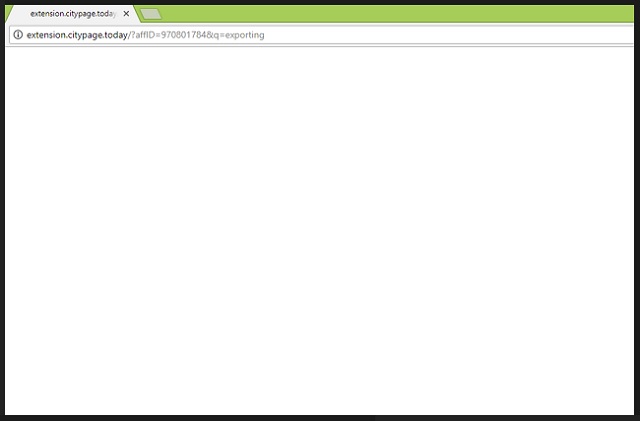The image showcases a rectangular box outlined with a black line, placed against a sage green background. At the top of the box, there is a white tab with the text "Extension City Page Today" written in bold, and an "X" icon positioned to the right of the text. Below this, within the box, there is a white circular icon containing an exclamation mark, indicating a warning or important note. Further down, the box features two horizontal grey lines, side by side. The screenshot does not provide any additional information about the content being exported or the context of the image.